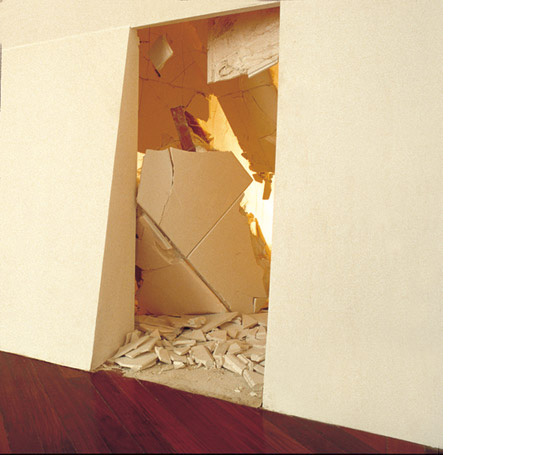The image is a photograph taken inside a ruined building. The interior shows walls that slant backward at an incline, covered in a vanilla ice cream color. The floor consists of dark redwood planks laid diagonally in the opposite direction of the walls. The focal point is an open doorway at the center of the image, where the door area is completely broken down with a variety of small rubble on the ground near the entrance and larger pieces scattered further in. The entrance's top part has a rectangular piece hanging down, and behind it, an 'N'-shaped structure seems to be falling toward the ground. Through the doorway, the next room appears in complete disarray with rubble made of broken tiles or concrete scattered everywhere. The ceiling has partially collapsed, leaving bits hanging down precariously. In the background, there's a very bright light that emphasizes the effects of a fire, but notably, there is no smoke visible.